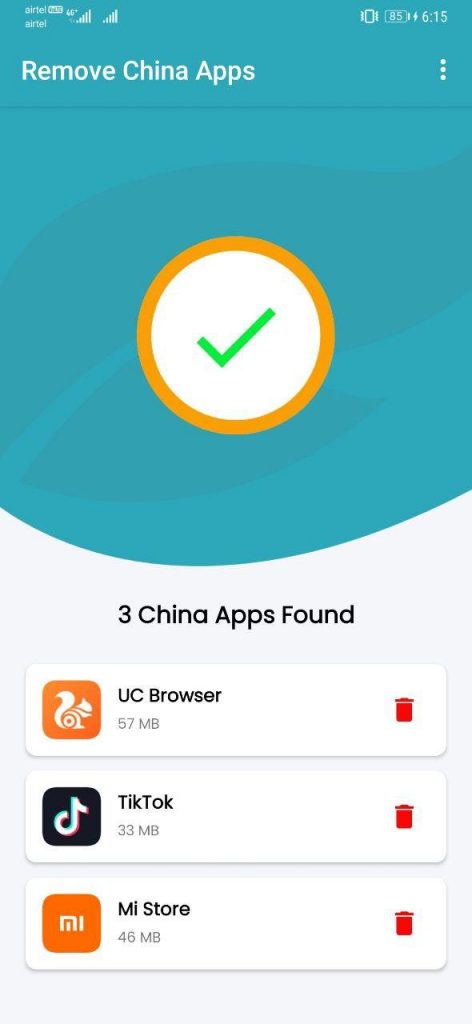A detailed description for the caption might be:

"This image shows a full screenshot of an Android phone displaying an app called 'Remove China Apps.' The app's interface features a prominent white background, with a section highlighted in aqua displaying the text '3 China Apps Found.' Listed below this, there are three specific apps identified for removal: UC Browser, Mi Store, and the highly popular social media app, TikTok. Each of these apps has a green checkmark next to it, indicating they can be removed. The screenshot also reveals the phone's status bar at the top, which shows a battery level of 85%, a time stamp of 6:15, and signal strengths for two different phone carriers, suggesting a dual SIM capability. The overall color palette is a mix of white, aqua, orange, and gray tones, adding a vibrant yet clean aesthetic to the app's interface. There is also some gray iconography in the background that is difficult to make out. This app hints at concerns over data privacy, especially with apps like TikTok, which is often scrutinized for data collection practices."